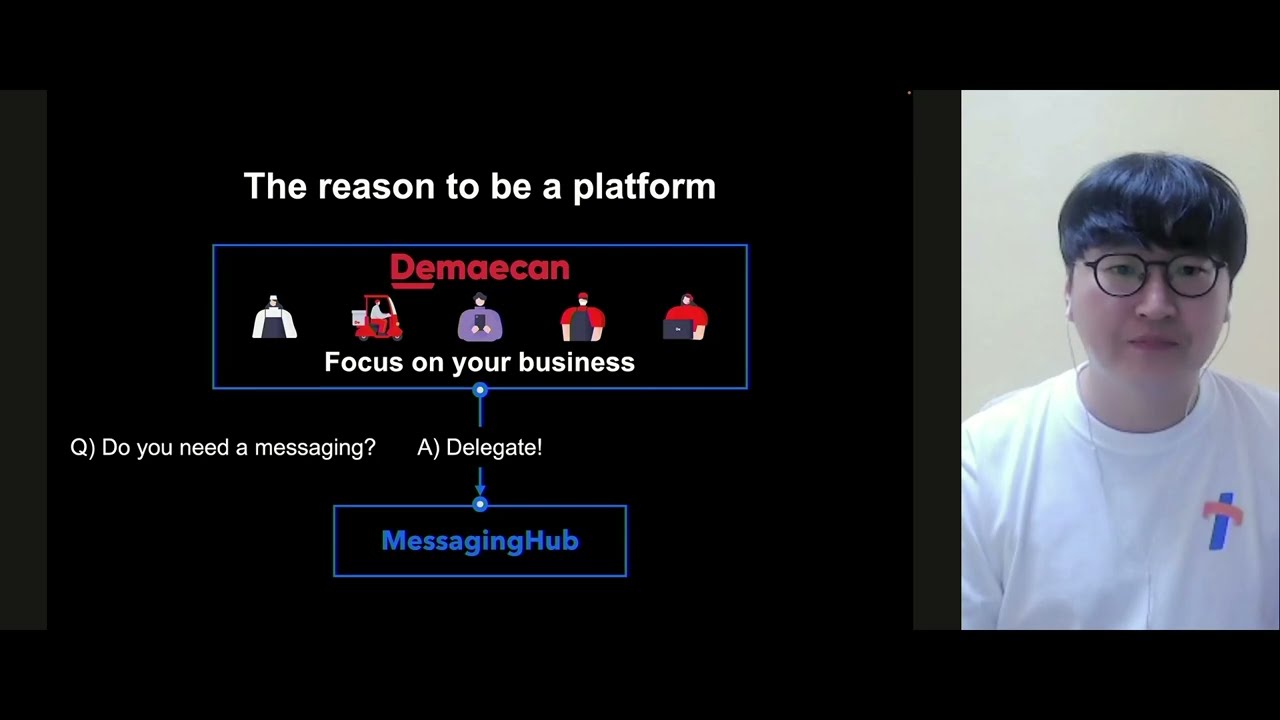The composite image is an artful blend of photography and digital editing, predominantly featuring a sleek black background. On the left side, spanning about two-thirds of the image, there is a promotional section with the following text elements in white: "the reason to be a platform." Below this, a blue outlined rectangle houses the red text "D'Macan" with a series of cartoon characters inside. These characters are dressed in red, white, and purple outfits, indicating various roles—one in white with a black apron, another driving a red forklift, and others in red shirts, hats, and black aprons. Further inside the rectangle, the phrase "focus on your business" is displayed in white text.

A blue vertical line beneath this section intersects with the phrase "Q (do you need a messaging) a (delegate!)" in white text. Further down, another blue-outlined rectangle contains the blue text "messaging hub."

The right third of the image shows an Asian man with a bowl cut and black hair, wearing black-rimmed glasses and white earbuds. He sports a white t-shirt featuring a blue and pink logo on the right side. The background behind him contrasts with a light brown color, which may vary slightly from beige to tan in different descriptions. The meticulous details of his expression reveal pink lips and a wide nose, adding a personal touch to the digitally amalgamated scene.